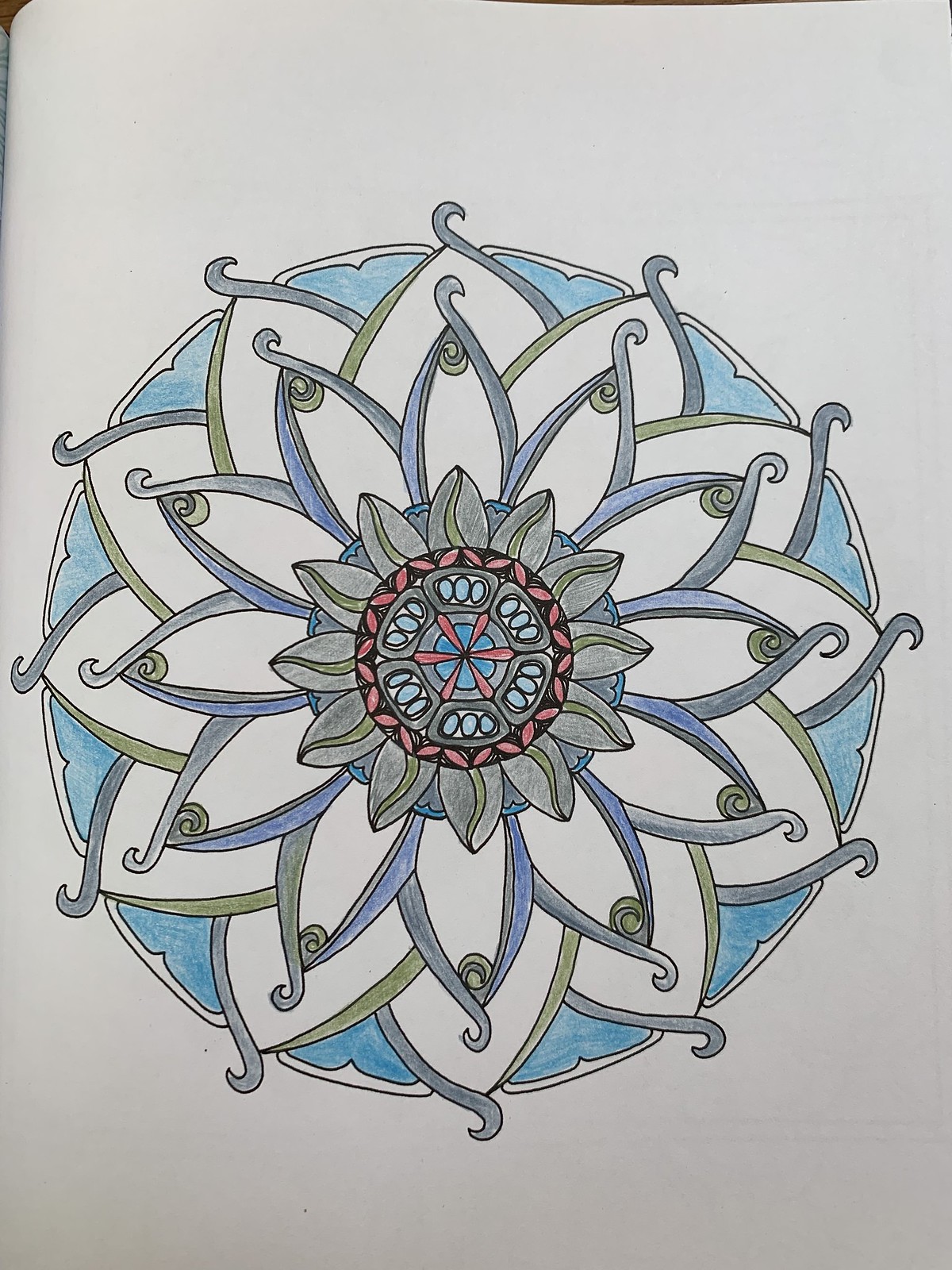A meticulously hand-drawn circular motif, reminiscent of traditional Celtic artwork, is displayed against a clean white paper background. The primary canvas is a soothing blue, accented by intricate patterns rendered in various shades of gray, blue, and green. These colors are skillfully intertwined to form Celtic knotwork that takes on a leaf-like, somewhat triangular shape. The circular design radiates outward in three or four concentric rows, culminating in vibrant red circles interspersed with additional blue and gray circular elements. These elements are artistically arranged in petal-like groupings, creating a harmonious and mesmerizing visual effect.